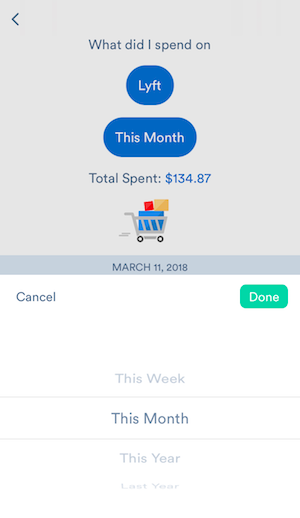The image displays the spending section of a budgeting app, possibly You Need A Budget or a similar application. The background at the top part of the screen is a very light gray, transitioning to a darker gray middle bar, and ending with a white lower section. 

In the upper left corner, there is a black left-arrow icon. Centrally positioned beneath it is the question, "What did I spend on?" Below this, a blue circle contains the word "Lift" in yellow text. Further down is a blue oval with the phrase "This Month" written in white font. Moving lower, the text "Total Spent" appears, followed by a figure in blue showing $134.87.

A gray shopping cart icon, appearing to move to the right, is pictured below this financial summary. The cart carries three boxes: a large blue box, a smaller red box stacked on top of it, and a slightly larger yellow box alongside.

On the darker gray line below the shopping cart, the date "March 11th, 2018" is displayed. To the left of this, the word "Cancel" is written in black text, while on the right, a green button with white text reads "Done."

Beneath these elements is a scrollable selection wheel allowing users to choose time frames like "This Week," "This Month," "This Year," and "Last Year," with "This Month" highlighted. Thin gray lines border the selected time frame at both the top and bottom.